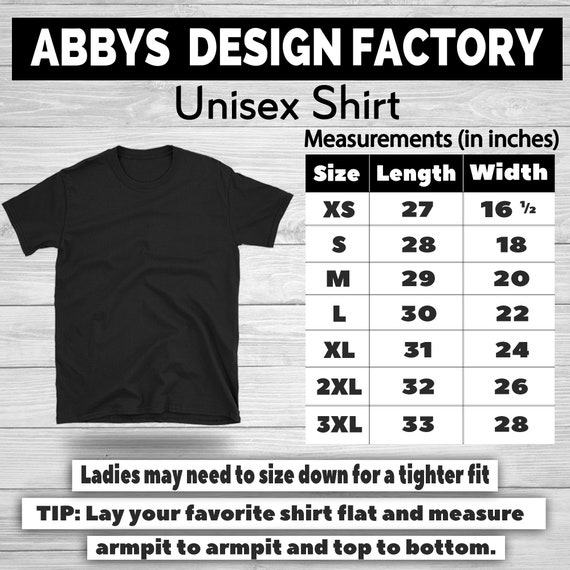The image is a detailed visual measuring chart for a black unisex t-shirt from Abbey's Design Factory. The backdrop consists of a light gray or off-white wall with horizontal wooden slats. At the top, a black banner prominently displays "Abbey's Design Factory" in white text. Below this, the black unisex shirt is centered on the left, accompanied by a measurement chart on the right, indicating sizes from extra small to 3XL. The measurements show lengths ranging from 27 to 33 inches and widths from 16.5 to 28 inches. At the bottom, three white banners with black text provide useful fitting tips, including a suggestion for ladies to size down for a tighter fit and a tip for measuring a favorite shirt flat from armpit to armpit and top to bottom.